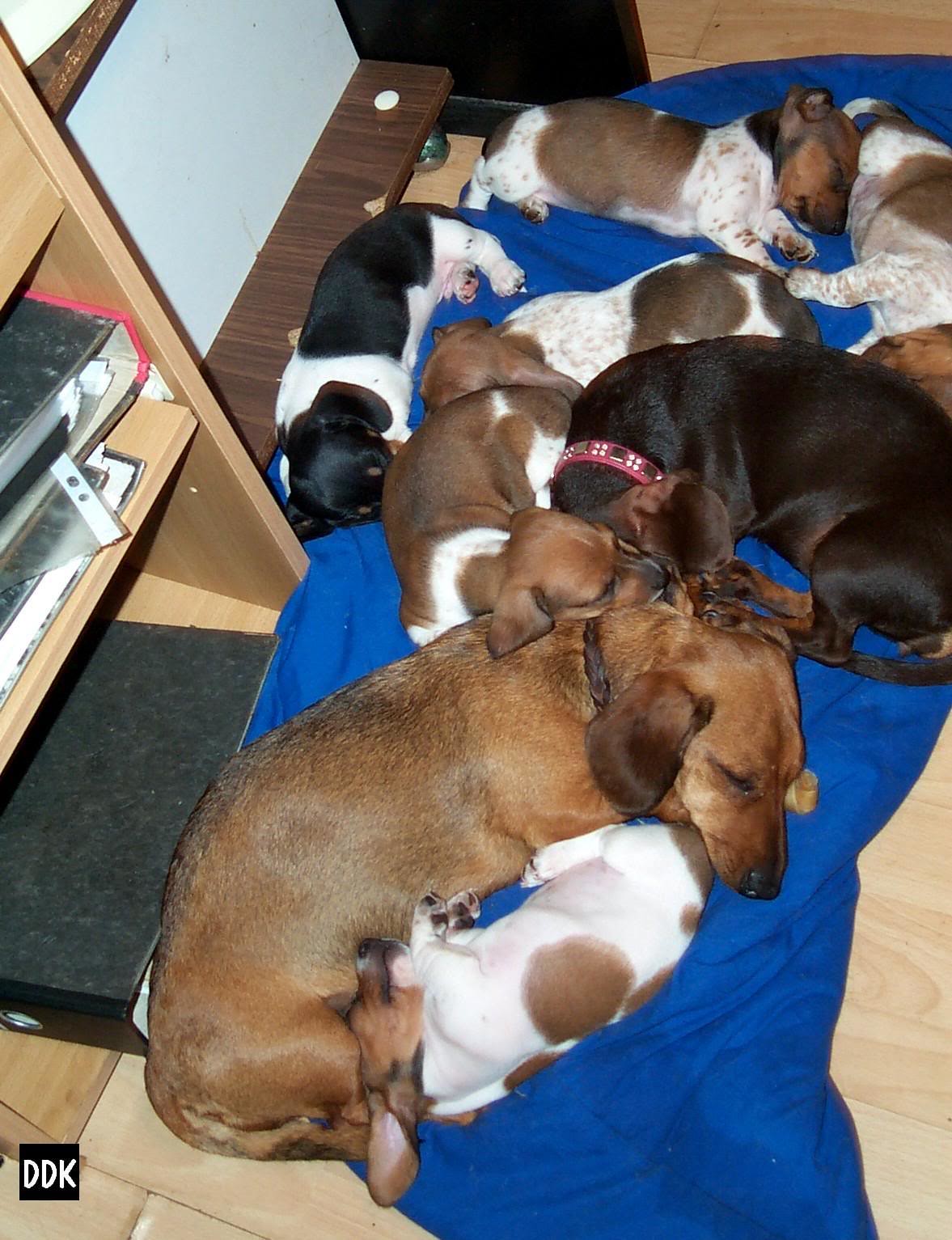The image showcases a heartwarming scene of a light brown mother dog and her seven puppies, all peacefully asleep on a soft blue blanket spread out on a light wood grain floor. Among the puppies, some are brown, some are brown and white, and one is black and white, all nestled closely together. Accompanying them is a dark brown dog with a shiny coat, donned with a red collar adorned with beads, while the mother dog wears a brown leather collar. They are situated in front of a somewhat disorganized set of beige wooden bookshelves that hold various books and binders, some visibly askew. On one side, a wooden slab juts out from the wall, possibly serving as an additional shelf. In the bottom left-hand corner of the image, the letters "DDK" are prominently displayed in bold, white font on a black rectangle.